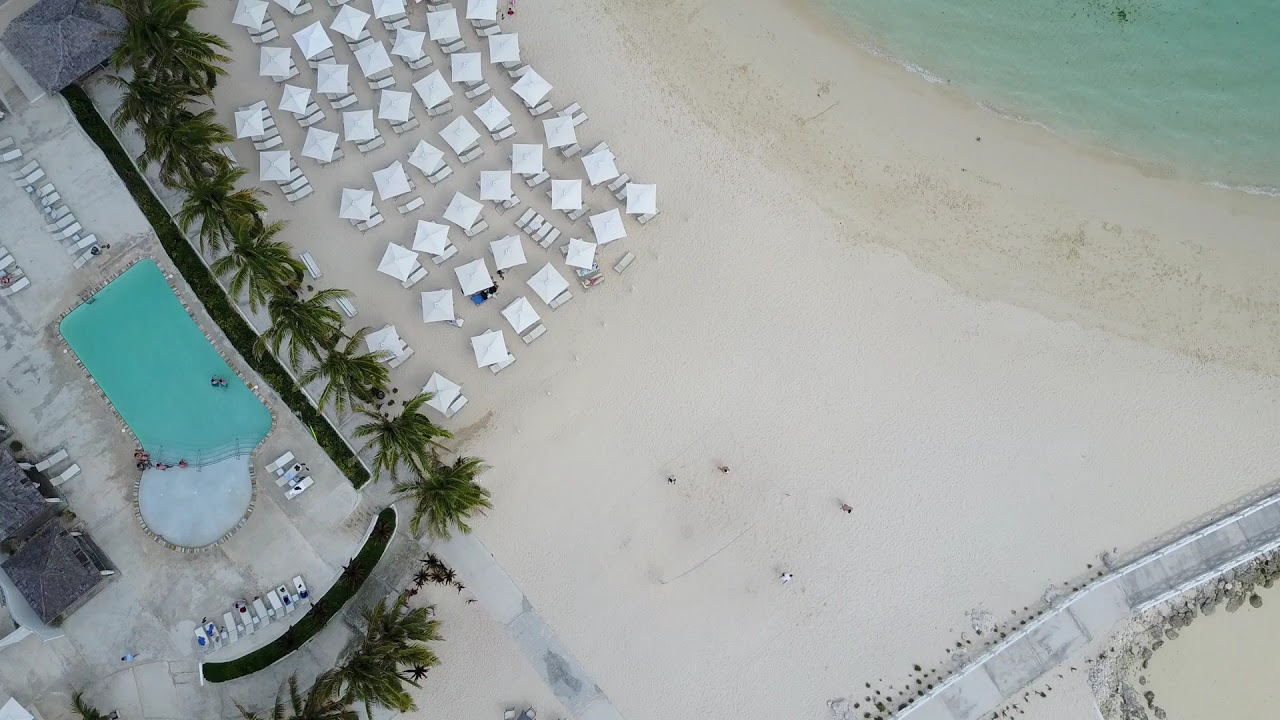This is a detailed aerial image looking straight down at a white sandy beach. In the upper right corner, the shoreline is visible with clear, light green aqua-colored ocean water. There is a slight stain on the sand where the water has reached. Moving to the left, there is a row of lounge chairs each shaded by white square umbrellas, arranged in a tidy line. Beyond these umbrellas, a row of lush green palm trees marks the boundary before a light green swimming pool. The pool features a semi-circle concrete platform at its bottom and a single person can be seen swimming in it. To the left of the pool, more lounge chairs are arranged in neat rows. At the bottom right of the image, a walkway runs along the sand with small sand patches sprinkled on it, bordered by barriers. Scattered throughout the beach and pool area are tiny figures of people, with about four or five visible walking or resting, adding life to this serene vacation spot.